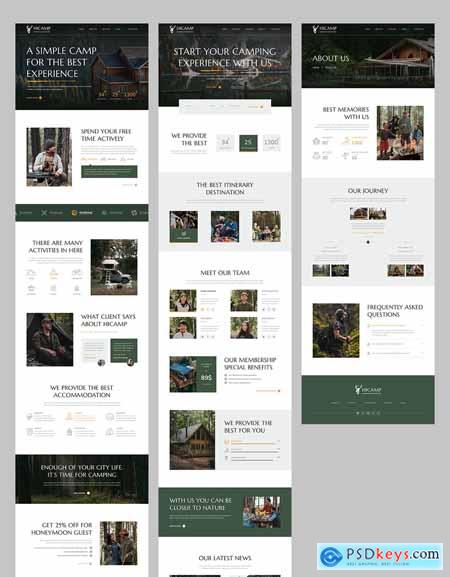This image, sourced from PSDKeys.com, features a distinctive light blue square label at the bottom right corner. This label is designed to resemble a button and includes an eye-shaped icon with a blue exterior and a white interior. The layout is divided into three vertical sections.

On the left section, a simple banner promotes "The Best Experience" for camping, accompanied by small, somewhat indistinct images of outdoor camping scenes. The center section invites viewers to "Start Your Camping Experience with Us" and showcases several images depicting various camping and outdoor activities. The right section is labeled "About Us," featuring another outdoor camping image to encapsulate the essence of the company's identity and offerings.